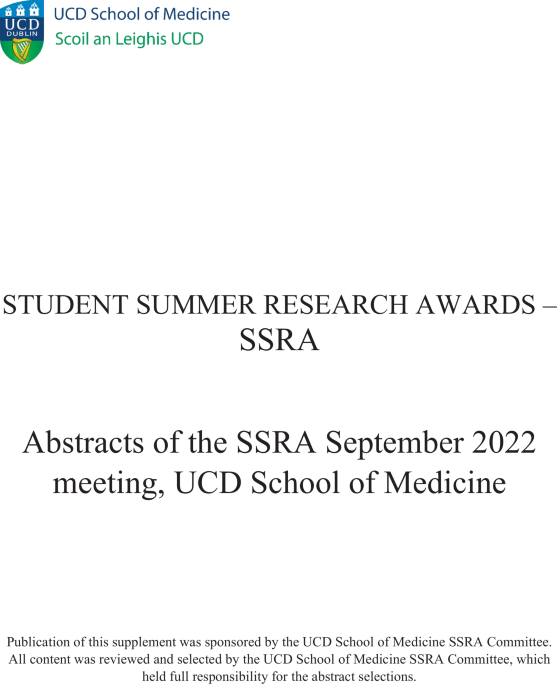This image features what appears to be the cover page of a publication or pamphlet from the UCD School of Medicine, likely in Dublin, Ireland. In the top left corner, there's a watermark of the UCD School of Medicine's logo. Adjacent to it, the text "Scoyle en Lais UCD" is displayed in green. The logo also appears on the left side, depicted as a shield with blue, dark blue, and green sections, and labeled "UCD Dublin." The title of the document reads "Student Summer Research Awards (SSRA)," followed by "Abstracts of the SSRA, September 2022." It is noted that the publication of this supplement was sponsored by the UCD School of Medicine SSRA Committee, which also reviewed and selected all the content, holding full responsibility for the abstract selections.